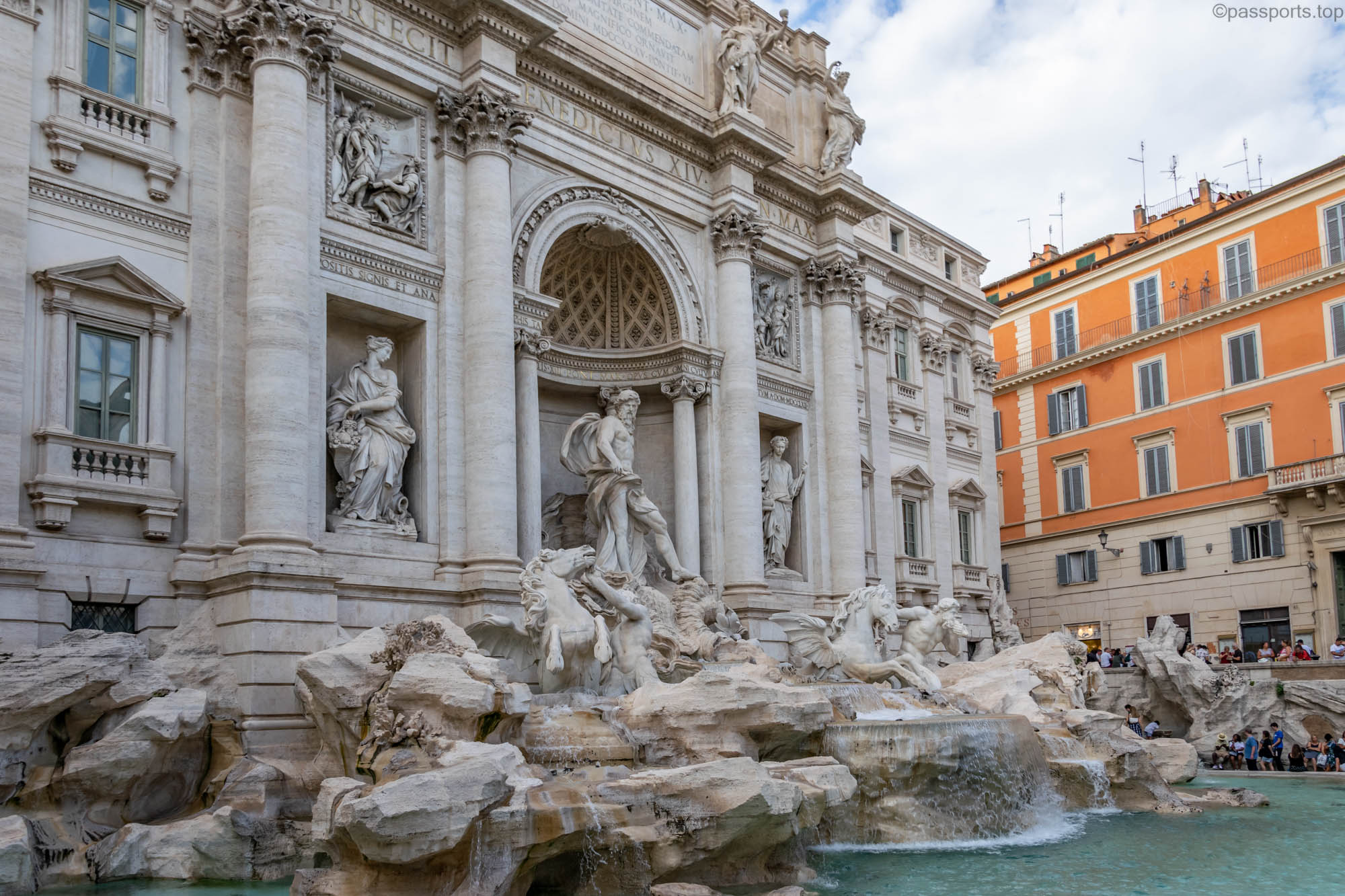This photograph captures an ornate architectural marvel by the water's edge, possibly taken in a place reminiscent of Venice or Greece. The main building, constructed with gleaming white stone, features a grand arched entryway adorned with a statue of a man draped in cloth standing atop a rocky formation. Surrounding this prominent figure, water cascades into a crystal-clear blue fountain. The front facade of the building showcases four white stone columns flanking the entrance, with intricate details along the stonework. Windows are prominently featured, framed by small, faux balconies carved into the building's sides, which include sculptures of draped women. Below the main sculpture, statues of men and horses, some appearing to wave, contribute to the fountain's grandeur. The water before the structure has a distinctive green hue. To the right, there is a large building with a cream-colored bottom half and an orange top half, adorned with numerous windows and gray shutters. The bright blue sky with white fluffy clouds frames the scene, adding to its picturesque quality. There are people milling about, adding life to this historic setting. In the top right of the photo, the text "passports dot top" is visible.